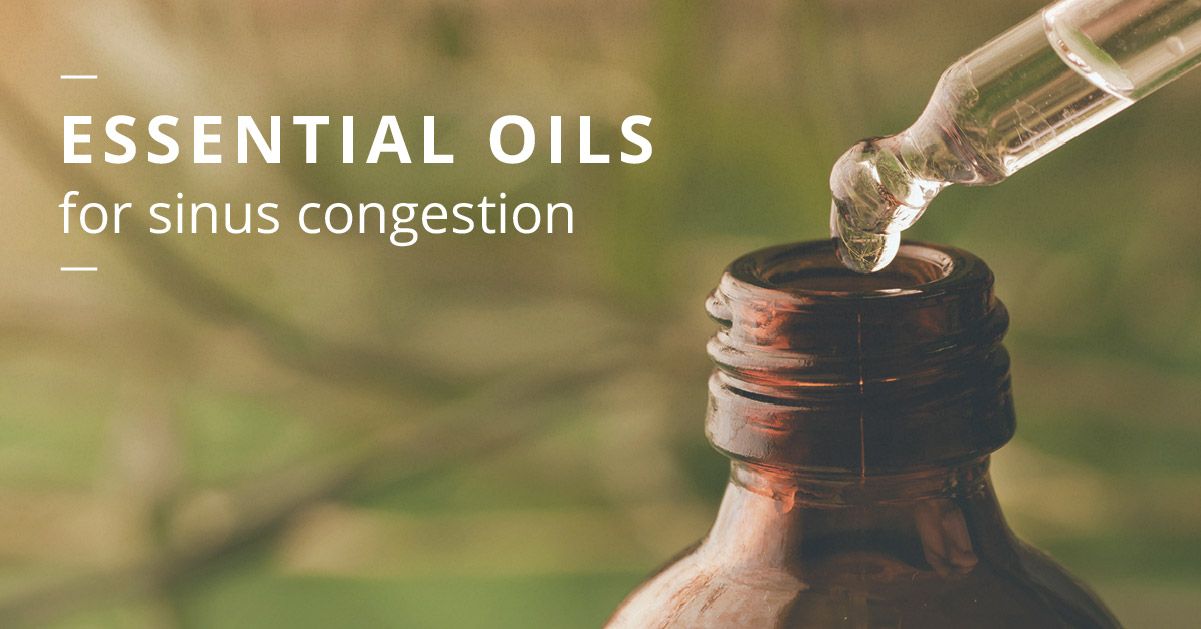The image depicts a close-up view of a deep amber-brown glass bottle with an open top, likely designed for a twist-on cap. Hovering above the bottle is a glass dropper filled with clear liquid, poised to release a drop into the bottle. The background is out of focus, featuring a mix of green and brown hues, offering a natural, earthy ambiance. On the left side of the image, white text reads "ESSENTIAL OILS" in all caps, followed by "for sinus congestion" in lowercase. The scene captures the precise moment a drop is about to fall from the dropper into the bottle, emphasizing the use of essential oils for sinus congestion relief.